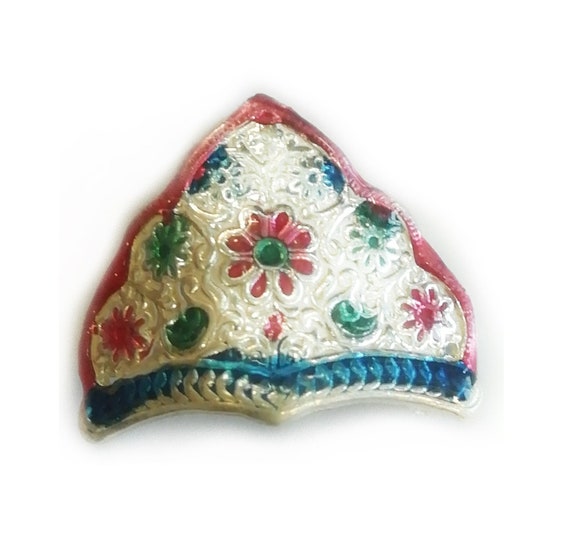The image showcases a finely detailed, triangular-shaped art object with a white background. The shape is slightly rounded at the top and scalloped at the bottom, resembling a tile or possibly decorated cake. The edges are adorned with intricate floral patterns, featuring a mix of pink, red, green, and blue flowers, some of which are in relief, allowing you to feel their textures. The focal point is a prominent red flower with a green center in the middle, flanked by smaller pink flowers and other vibrant floral arrangements along the top edges resembling a scalloped border. The bottom of the object has a braided pattern painted blue and white. The left and right sides of the object have a red trim, while the overall finish indicates meticulous yet somewhat imperfect craftsmanship, with some paint spilling outside the lines. The entire object exudes a colorful, tactile, and intricately detailed design, making it the centerpiece of the picture.